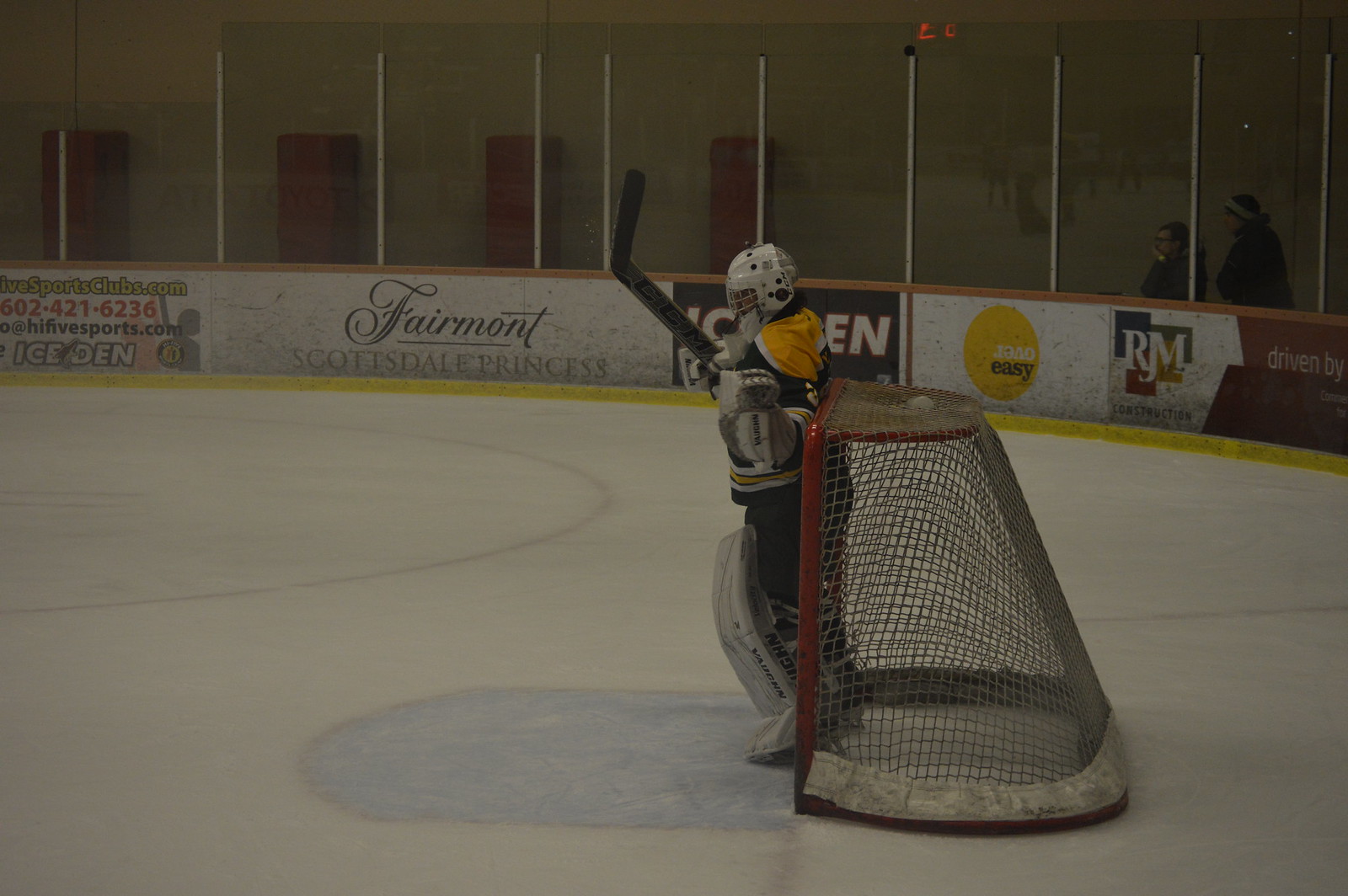The image captures the interior of a dimly lit ice hockey arena, focusing on a goalie. The ice, white with red lines and a blue half-circle in front of the net, clearly identifies the setting. The goalie is positioned in front of a red net, facing left, providing a side view. He is fully equipped with protective gear, including a white helmet and a distinctive black, yellow, and white jersey. His goalie stick is raised above his head. The background features a wall covered halfway with advertisements, including notable ones such as Fairmont Scottsdale Princess and Ice Den, with the upper half made of plexiglass. There are also two audience members visible to the right behind the goalie, along with red barriers and a possible exit sign at the top.